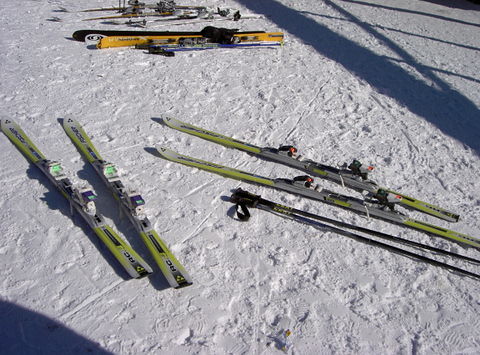This color photograph, taken outdoors during the daytime on a ski slope, showcases multiple pairs of skis laid out on hard-packed snow with visible footprints and ski marks. In the foreground, there are two prominent pairs of skis. The pair on the left is olive green, while the pair on the right is light yellow with black writing, both featuring bindings. There is also a pair of black ski poles with wrist loops next to them. Further back in the image, more skis are scattered on the snow, including a bright yellow pair with black bindings and another pair that is light orange with black writing. Angular shadows stretch across the snow, adding a contrast to the scene, although their source is unclear, possibly a bridge. The photograph captures the stillness and scattered equipment typical at the base of a ski hill, devoid of people or text.